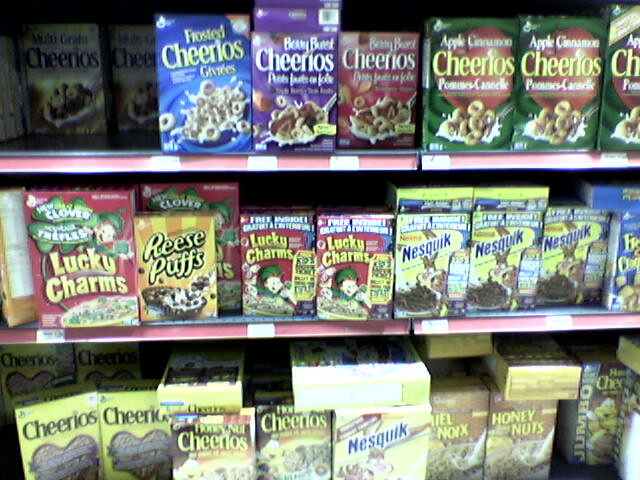The image depicts a well-organized grocery store shelf dedicated to breakfast cereals. There are three metal shelves, each lined with a red rim and showcasing a variety of cereal brands. The top shelf displays an assortment of Cheerios boxes, each in brightly colored packaging. There’s a box of Frosted Cheerios with a blue background, Berry Blast Cheerios in both purple and red backgrounds, and Apple Cinnamon Cheerios with a green and red background. The middle shelf holds boxes of Lucky Charms, Reese's Puffs, and a Nesquik cereal, suggesting a mix of popular and chocolate-infused breakfast options. The bottom shelf features some classic cereal varieties, including the original Cheerios in their iconic yellow box, Honey Nut Cheerios, and an assortment of Off Brand Cheerios. In front of each product are little white price tags, indicating the cost of the items. The arrangement of the products provides a visually appealing and accessible selection for shoppers looking to start their day with a hearty breakfast.